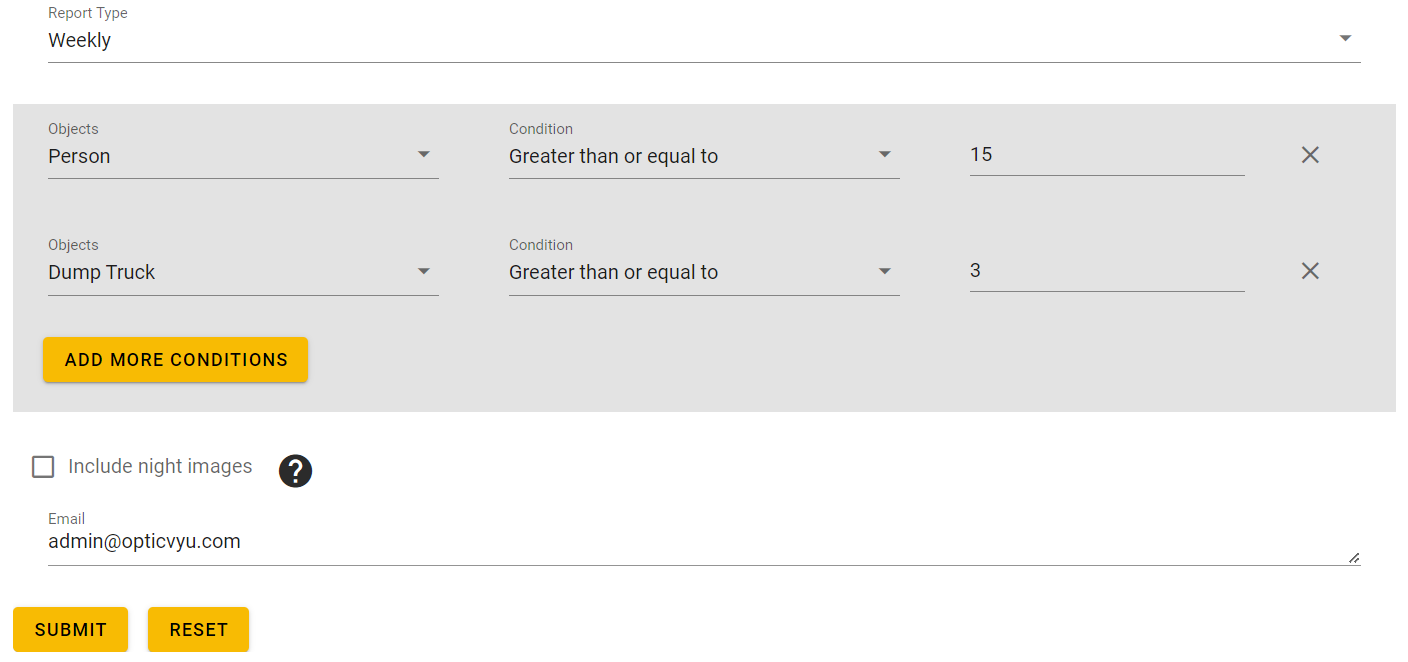This screenshot showcases a segment of a website's user interface, specifically focusing on a report configuration section. The visible portion of the site allows the user to select various report parameters. Currently, the "Report Type" option is set to "Weekly." 

The interface features criteria-based selections where the primary criterion appears to be a "person" object, which is stipulated to be greater than or equal to 15. Additionally, a secondary criterion involves "dump truck" objects, set to be greater than or equal to 3—this number is lesser than the one specified for the "person" object.

An option for including night images is present but remains unselected by the user. Below this, an email address has been provided, likely for administrative purposes or for receiving additional data. The email address specified is "admin@opticvyu.com," presented in a small text box towards the bottom of the section.